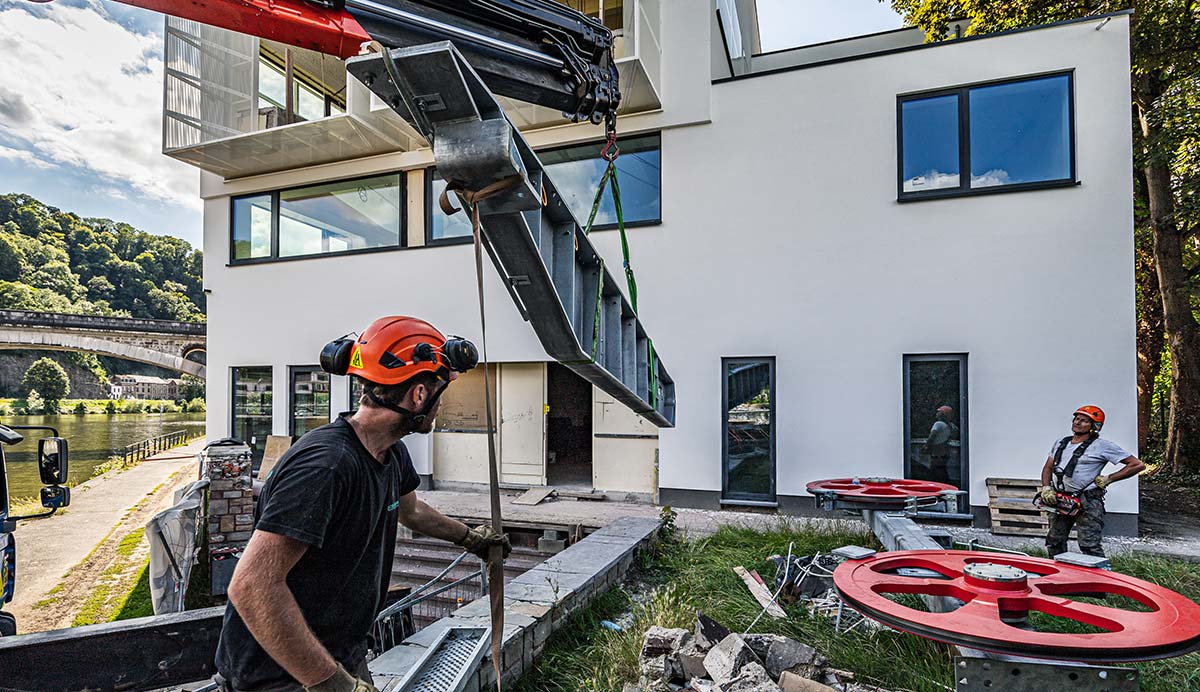This image depicts a construction site for a large white house or residential building situated near a pond or river, with a bridge and dense trees visible in the background. The multi-story house has a notable arrangement of windows, including three large rectangular ones on the top and several window-like openings on the lower level near the unfinished doors. Two construction workers are in action: one near a large machine with oversized, cutout orange wheels, and another on what appears to be scaffolding. Both workers are wearing orange hard hats, with one in a black shirt facing away from the camera and another in a gray shirt, slightly farther away, facing towards the camera. The gray-shirted worker also has a tool belt draped around his neck. The scene blends typical construction elements with some ambiguous features, like peculiar large reels that add an enigmatic touch to the worksite.